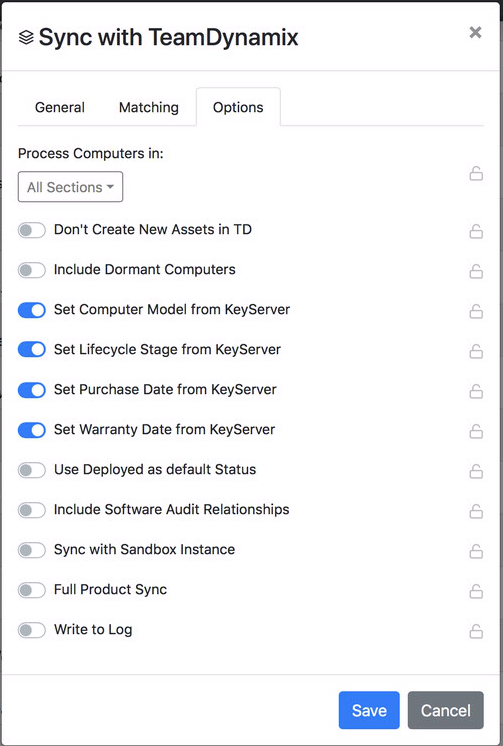The image features a rectangular interface with a black outline and an off-white background. At the top, in black text with a pink corner, it reads "S, Y, and Z's are synced with Team Dynamics." On the right-hand side, there is a gray 'X' symbol followed by a horizontal gray line.

Below, in black text, the categories "General," "Matching," and "Options" are listed. The "Options" category contains the following settings presented in a list format:

1. A gray oval next to "Don't Create New Assets in TD".
2. A gray oval next to "Include Dormant Computers".
3. A blue oval next to "Set Computer Model for Key Server".
4. A blue oval next to "Set Lifecycle Stage from Key Server".
5. A blue oval next to "Set Purchase Date from Key Server".
6. A blue oval next to "Set Warranty Date from Key Server".
7. A gray oval next to "Use Deploy as Default Status".
8. A gray oval next to "Include Software Order Relationships".
9. A gray oval next to "Sync with Sandbox Instance".
10. A gray oval next to "Full Product Sync".
11. A gray oval next to "Write to Log".

At the bottom, there are two buttons: a blue button labeled "Save" and a gray button with white text labeled "Cancel".

In summary, the settings toggle between on (represented by blue ovals) and off (represented by gray ovals) to control synchronization and workflow options related to computer assets and key server interactions.